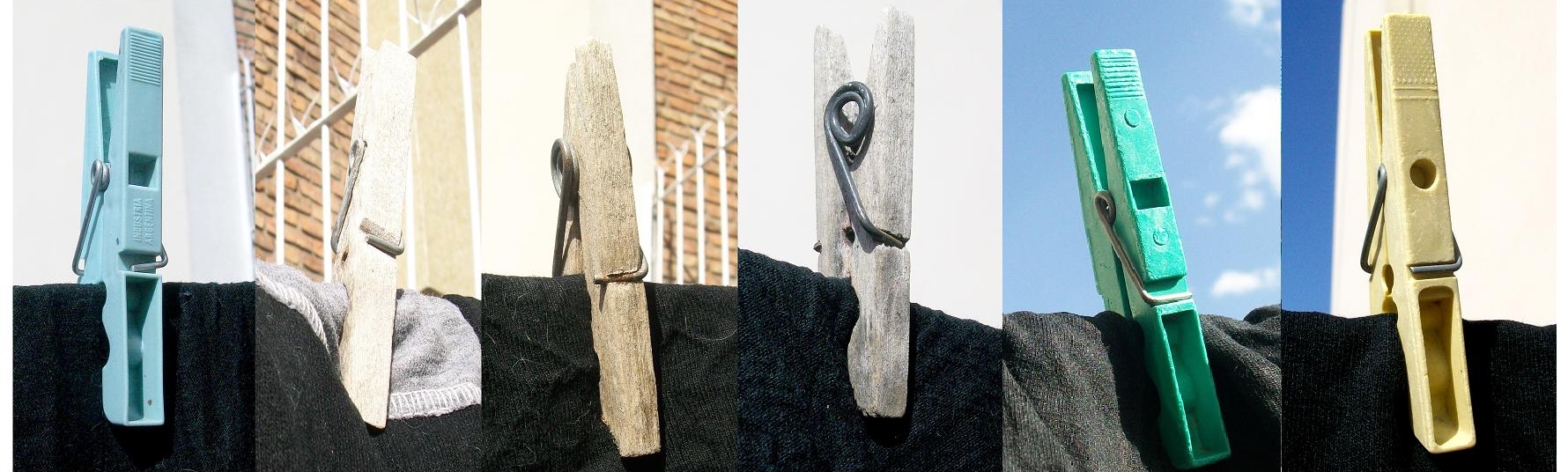This composite landscape-format image is made up of six individual photographs, each featuring a close-up of a clothes pin holding a dark piece of clothing on a line. Starting from the left, the first photograph showcases a blue plastic clothes pin against a white background, holding a black item. The second image features a wooden clothes pin gripping a dark grey and black item against a backdrop of red brick and a security gate. In the third image, an older wooden clothes pin holds a black item, with a background showcasing white wool and more red brick featuring a security gate. The fourth image presents another vintage wooden clothes pin holding a black item against a white background. The fifth photo displays a bright turquoise plastic pin, similar in style to the first pin, clamping a dark grey item against a backdrop of blue sky dotted with white clouds. The final, far-right image includes a yellow plastic clothes pin of a different design securing a black item, set against the backdrop of a white building and a segment of dark blue sky.